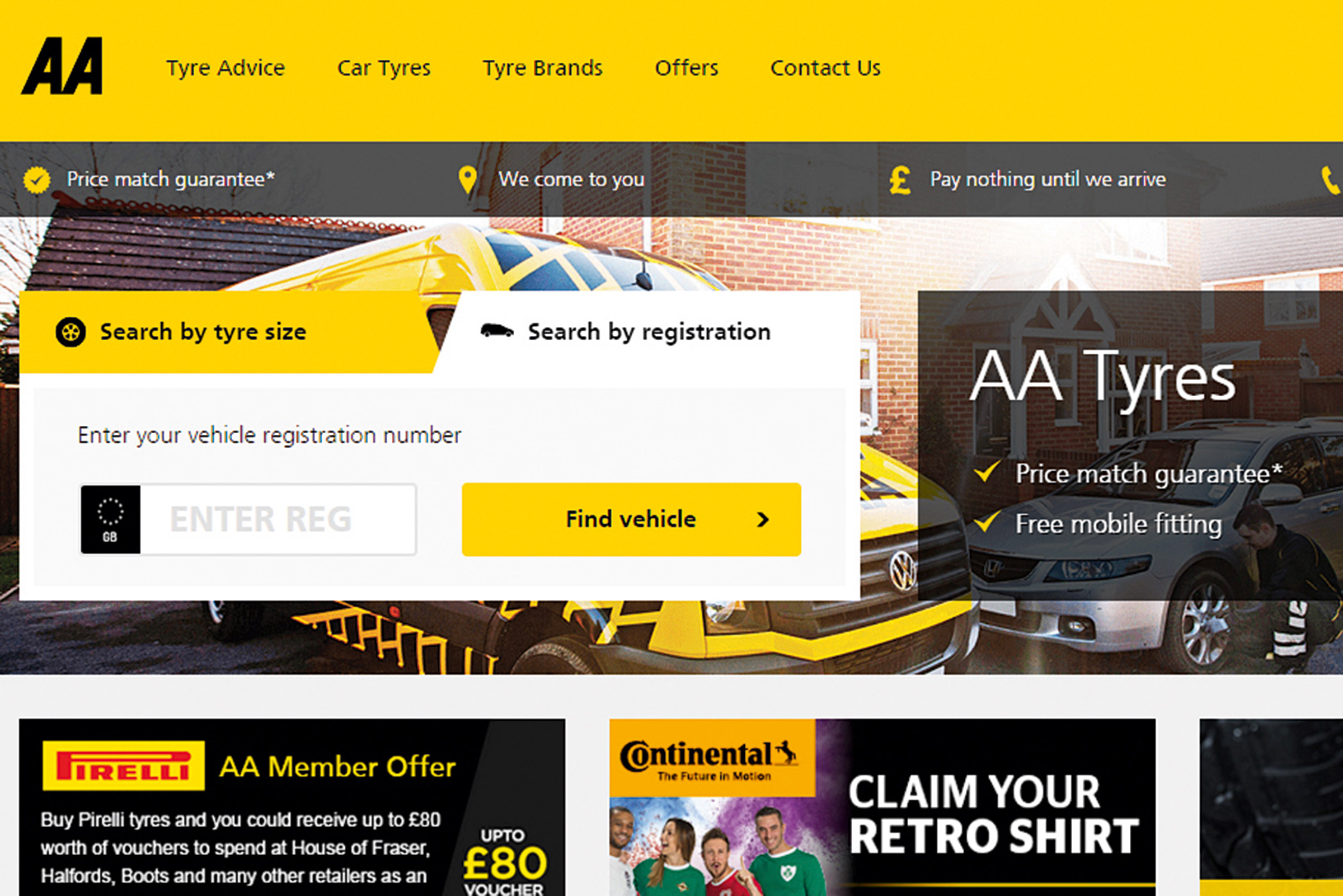The image displays a homepage for AA's website, focused on tire services. At the top, a yellow-orange bar with black lettering features "AA" in italicized capital letters on the far left. To the right of it are menu options including "Tyre Advice" (with "Tyre" spelled T-Y-R-E), "Car Tyres," "Tyre Brands," "Offers," and "Contact Us."

Beneath this, a dark gray, partly transparent bar holds white-font text offering "Price Match Guarantee" (marked with an asterisk), "We Come to You," and "Pay Nothing Until We Arrive," each accompanied by small yellow icons on their left.

Dominating the central background, a photograph shows part of a van with blue, yellow, white, and black markings, bearing the Volkswagen emblem on the grille. To the right of the van, a silver car is parked with a man standing next to its tire. In the backdrop, a brick building is visible.

On the left-hand side, a vertical rectangular tab provides search options. An orange tab labeled "Search by Tyre Size" sits above a white tab stating "Search by Registration," the latter appearing selected. Below this, a light gray box prompts users to "Enter your vehicle registration number," with a white command prompt. An orange-yellow button to the right reads "Find Vehicle" in black text.

On the front right side, a dark gray, partially transparent rectangle announces "AA Tires Price Match Guarantee Free Mobile Fitting."

At the bottom of the image, three rectangles feature various offers: one for Pirelli with an "AA Member Offer," another for Continental, and a third advertising "Claim Your Retro Shirt." These rectangles are primarily dark gray or black with additional text, set against a light gray background. A fourth rectangle, partially visible, is also present.